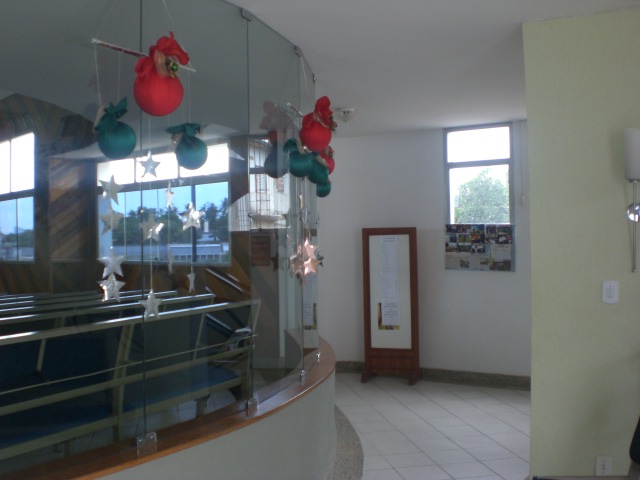The image reveals an indoor setting featuring a countertop with a wooden top positioned against white walls. From the ceiling hang silver stars on silver strings, alongside three bags—one red and two in a bluish-green color. The room has white tile floors and a white ceiling. On the back wall, below a window, there is a pin board with various images or photos, and a smaller wooden billboard with a paper on it stands to its left. The right side hosts an off-white wall with a light switch. To the left, a large glass divider encloses an area furnished with blue and chrome benches, suggesting it might be a general venue for gatherings, possibly a church or a meeting space. The decor, featuring hanging bags and stars, suggests a festive or event-related purpose.